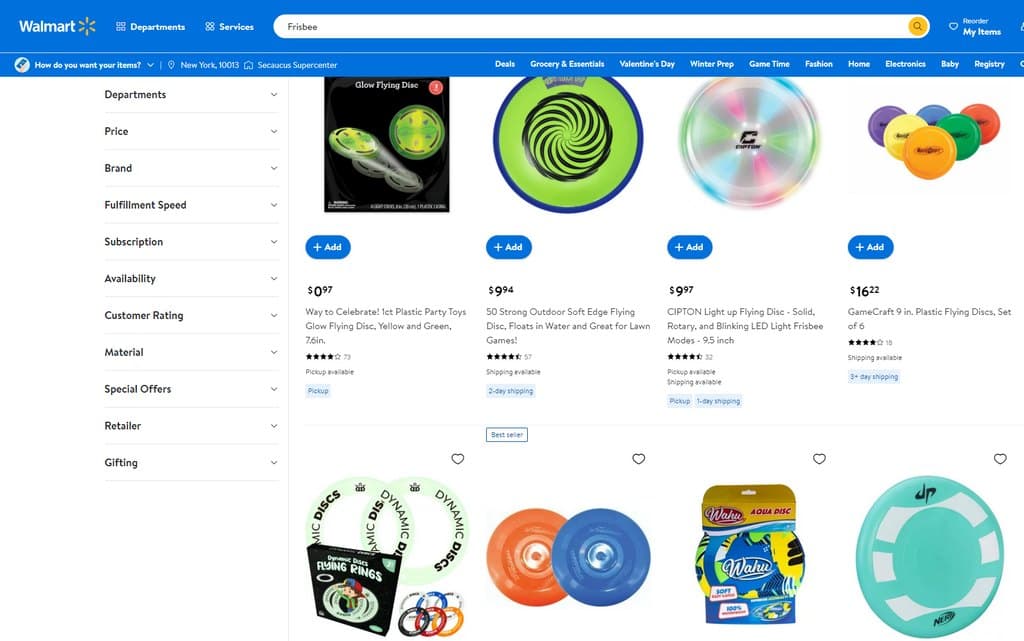Screenshot Overview of Walmart.com - Frisbee Section

The screenshot showcases the Walmart.com interface, specifically focused on Frisbee products, with multiple layers of navigation and product listings.

### Top Navigation Bar:
- **Blue Banner:** Occupying the very top of the screenshot.
- **Walmart Logo and Name:** Positioned on the far left.
- **Links:** Includes 'Departments' and 'Services' to the right of the logo.
- **Search Bar:** An elongated, oval search bar with 'Frisbee' on the left side and a yellow magnifying glass icon on the right.
- **Additional Options:** Next to the search bar are a heart icon and a 'Reorder My Items' link.

### Lower Sub-navigation (Still within Blue Banner):
- **Icon:** Depicts a hand holding a book.
- **Text:** Reads, "How do you want your items," followed by a dropdown menu.
- **Location:** Displays "New York, NY 10013" with a house icon labeled "Secaucus Supercenter."
- **Categories:**
  - Deals
  - Grocery and Essentials
  - Valentine's Day
  - Winter Prep
  - Game Time
  - Fashion
  - Home
  - Electronics
  - Baby
  - Registry

### Left-Side Vertical Filters:
- **Filter Categories:**
  - Departments
  - Price
  - Brand
  - Fulfillment Speed
  - Subscription
  - Availability
  - Customer Rating
  - Material
  - Special Offers
  - Retailer
  - Gifting

### Product Listings:
Eight Frisbee-related products are displayed in two rows.

#### First Row:
1. **Glow Flying Disc:**
   - **Image:** Yellow and green glowing disc in a black square.
   - **Price:** $0.97
   - **Description:** Way to Celebrate, 1 count, plastic party toys, 7.6 inches.
   - **Rating:** 7.3 stars
   - **Availability:** Pickup available.
   
2. **Green, Black, and Blue Frisbee:**
   - **Price:** $9.94
   - **Description:** 50 Strong Outdoor Soft Edge Flying Discs, floats in water, great for lawn games.
   - **Rating:** 5.7 stars
   - **Availability:** Shipping available (Two-day shipping option).

3. **Multicolored Frisbee with 'Cipton' Logo:**
   - **Price:** $9.97
   - **Description:** Cipton Light Up Flying Disc, solid, rotary, and blinking LED light modes, 9.5 inches.
   - **Rating:** 4.5 stars from 52 reviews.
   - **Availability:** Pickup available, shipping available (One-day shipping option).

4. **GameCraft 9-inch Plastic Flying Discs (Set of 6):**
   - **Price:** $16.22
   - **Description:** Includes six multicolored discs arranged in a triangular pattern.
   - **Rating:** 4 stars from 18 reviews.
   - **Availability:** Shipping available (Three-plus day shipping option).

#### Second Row:
1. **Dynamic Discs Flying Rings:**
   - **Image:** Only, no description provided.

2. **Orange and Blue Frisbees:**
   - **Image:** Only, no description provided.

3. **Wahoo Aqua Disc:**
   - **Image:** Multicolored disc with a floral pattern.
   - **Image:** Only, no description provided.

4. **Teal Frisbee with Nerf Logo:**
   - **Image:** Only, no description provided.

This detailed account gives a comprehensive look at the layout and contents of the Walmart.com screenshot featuring Frisbee products and the navigational elements included.